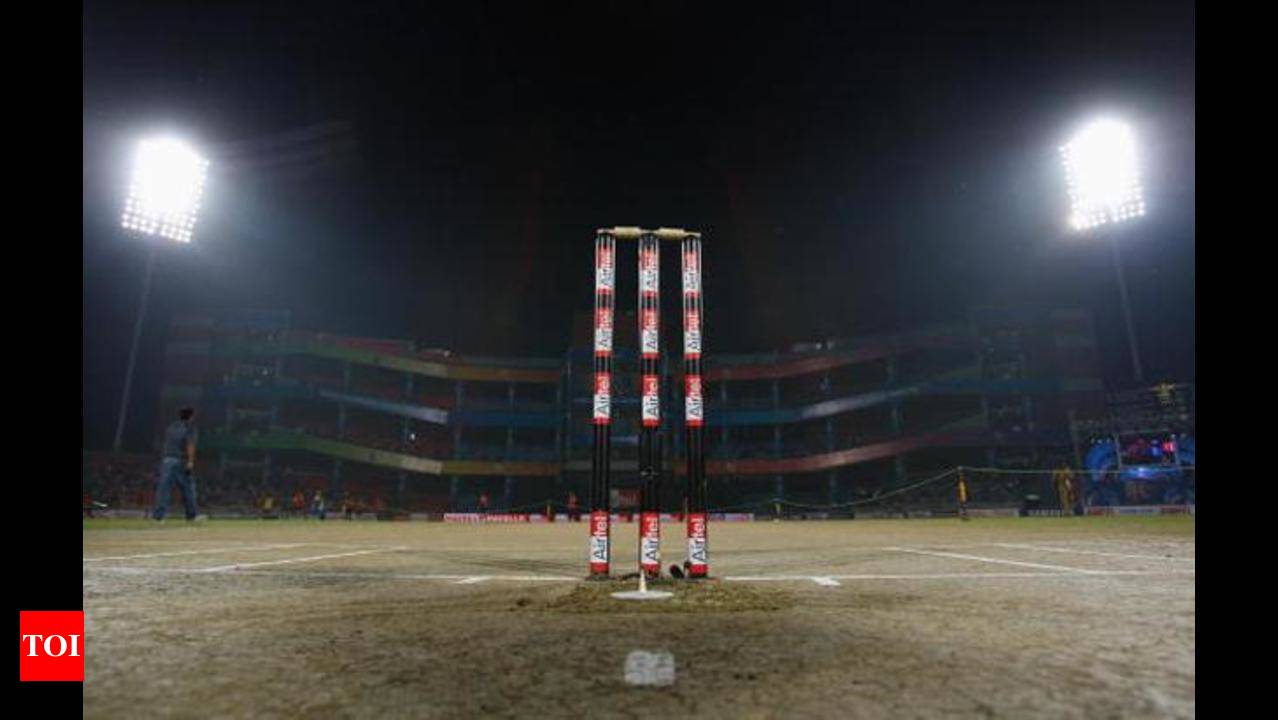The photograph captures a night scene in a cricket stadium. The horizontally rectangular image features a green playing field prominently in the center. At the heart of the field is a wicket, comprised of three stumps colored red, black, and white, with a single horizontal bail perched on top. To either side of the field are two large, bright floodlights casting their glaring light towards the center of the stadium. In the background, there are stands adorned in red, blue, and yellow, filled with spectators.

The overall setting appears outdoors, with a black night sky overhead and artificial lighting illuminating the scene. The left and right edges of the photograph are bordered by a black pattern, making the internal image appear square. Inside the left border, there is a red square with white lettering spelling out "T-O-I." Spotlights positioned in the upper corners further emphasize the nighttime atmosphere. 

A few players can be seen walking on the field, with one player in a blue uniform standing out towards the left side of the image. The composition suggests that the camera is positioned almost at ground level, emphasizing the height of the stumps and the structure of the stadium. There are various advertisements and white signage visible around the field, adding to the lively and commercial nature of the sporting event.